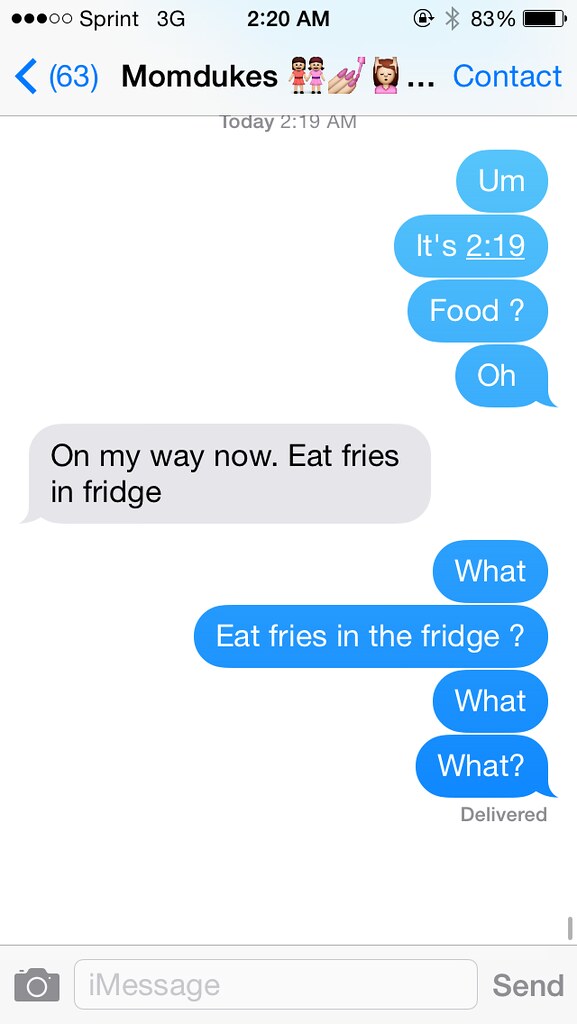The image is a detailed screenshot of a texting conversation on an iPhone. At the top of the screen, it indicates the carrier 'Sprint', the time '220 AM', 3G network status, and the battery life at '83%'. The contact name displayed is 'Mom Dukes', and the timestamp reads 'Today at 2:19 AM'. The conversation shows blue text bubbles from the phone's owner on the right side, and gray text bubbles from 'Mom Dukes' on the left side. 

The text in the blue bubbles reads sequentially:
1. "It's 2:19. Food?"
2. "Oh."
3. "What? Eat fries in fridge? What? What?"

The gray bubble responds to the first message with:
1. "On my way now. Eat fries in fridge."

At the bottom, there's an input field for typing a new message, with a small camera icon to its left and a send button on the right. The white background of the screen ensures that the text stands out clearly. The entire conversation ends with a delivery status saying "Delivered."